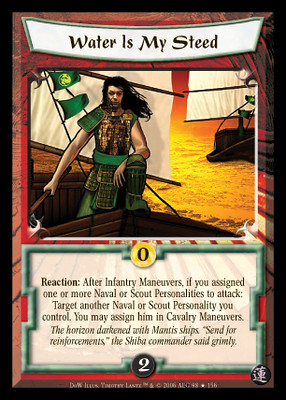The image depicts a beautifully illustrated rectangular card, seemingly from a card game akin to Magic: The Gathering. The card features the artwork of a character dressed in medieval-style green armor, complete with shoulder pads, standing confidently on a boat with a sail. The character wields either a staff or an axe, and notably lacks a helmet. Behind the character is an expansive scene of golden-yellow water, indicating an ocean, with another ship visible on the horizon. Green flags adorn the boat, one of which has a yellow logo.

At the top of the card, there's a banner that reads, "Water is my steed." The card includes detailed text, starting with "Reaction, after infantry maneuvers: If you assign one or more naval or scout personalities to attack, target another naval or scout personality you control. You may assign him in cavalry maneuvers." Additional narrative text mentions a commander grimly ordering reinforcements, and there are notable elements such as a number two in a circle, a zero in a yellow circle, and a predominantly brown border with some red accents.